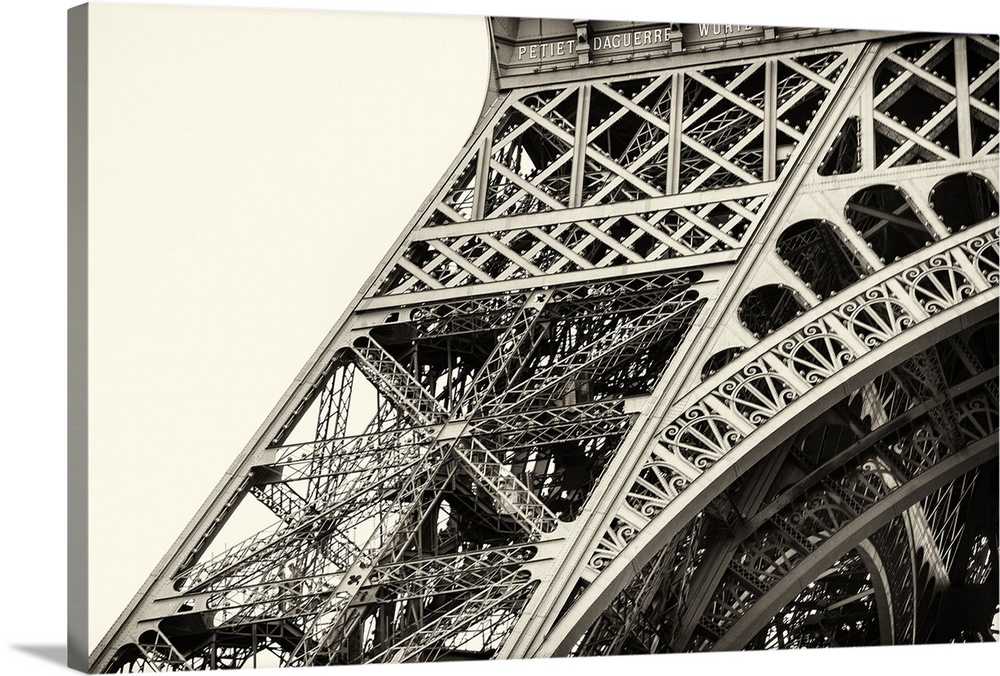This black and white vintage sepia-toned image captures a close-up of the mid-lower portion of the Eiffel Tower, showcasing its intricate metalwork. The photograph focuses on the intricate girder work and steel crosshatching that form the tower's structure, with beams and struts intersecting diagonally, horizontally, and vertically. The image includes a partial view of the lower arch and is dominated by the detailed web of metal, giving it a somewhat chaotic appearance. The shot is zoomed in, filling roughly three-quarters of the frame with the tower's metal framework, and includes some French lettering at the upper part of the image that reads, "Pitié Daguerre." There are no people, vegetation, or animals present, enhancing the focus on the architectural details.